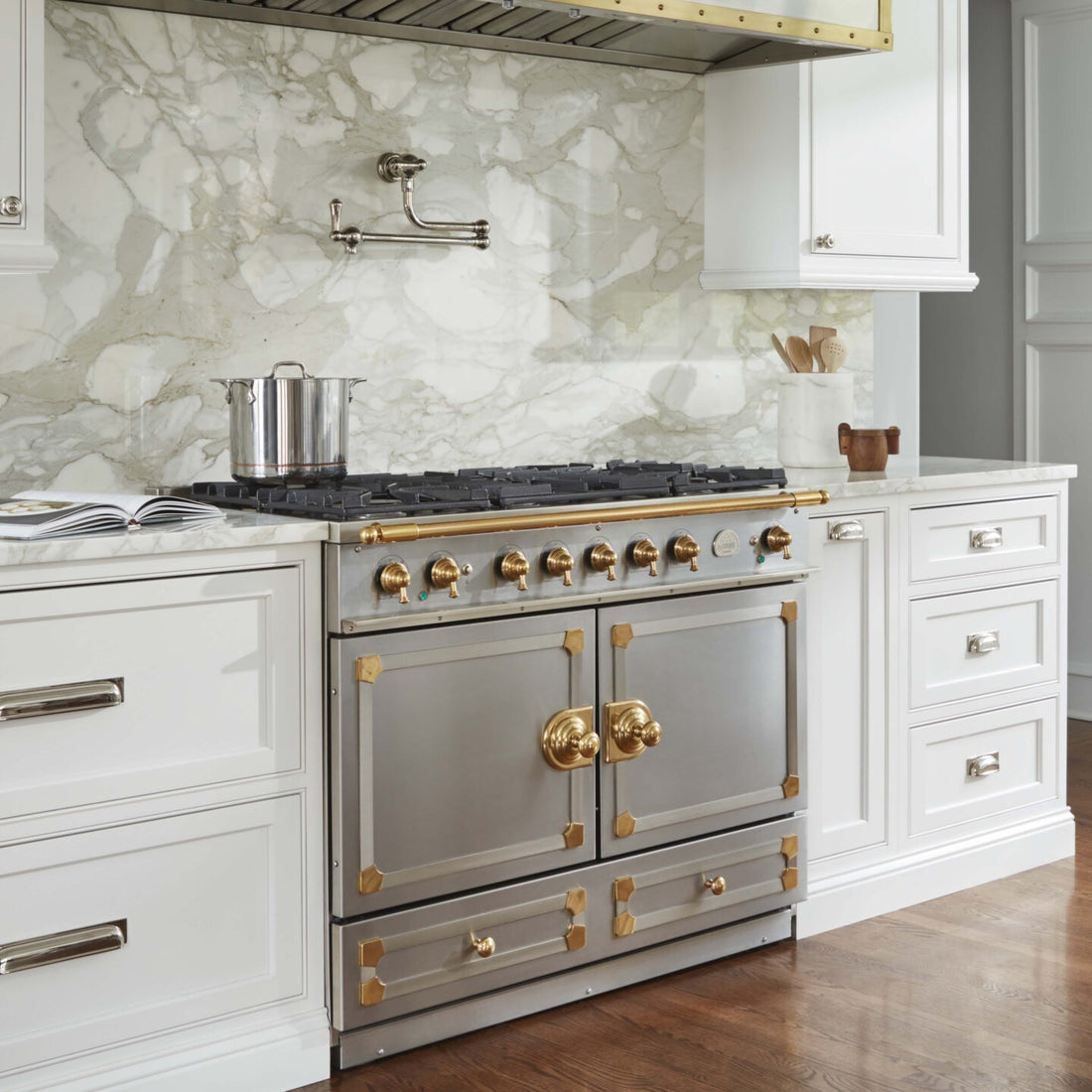The photograph, taken indoors, captures an immaculately pristine and luxurious kitchen. Central to the image is a large, stainless steel, 8-burner gas stove, under a substantial stainless steel hood. The stove, which appears almost commercial yet elegant, features a raised grill top suitable for lighting propane or natural gas beneath it. It is adorned with gold or brass knobs along the front and a small gold rail for hanging towels. Unique to the stove are its double oven doors, which open outward like cupboard doors, complemented by two drawer handles at the bottom that suggest additional storage or a warming drawer. On the back left burner sits a large stainless steel pot.

The surrounding countertop is a light white and gray marble that seamlessly continues into the matching marble backsplash behind the stove, lending a cohesive, sophisticated look to the space. Adding to the functionality and luxury is a water spout mounted on the backsplash, allowing for pots to be filled directly on the stove. Above the stove, additional cabinetry provides storage, with white cabinets framing the hood on both the left and right sides. The lower cabinets beneath the countertop are also white, fitted with sleek stainless steel handles. The kitchen floor transitions from the lower right-hand corner with a wooden texture, further enhancing the kitchen's elegant aesthetic.